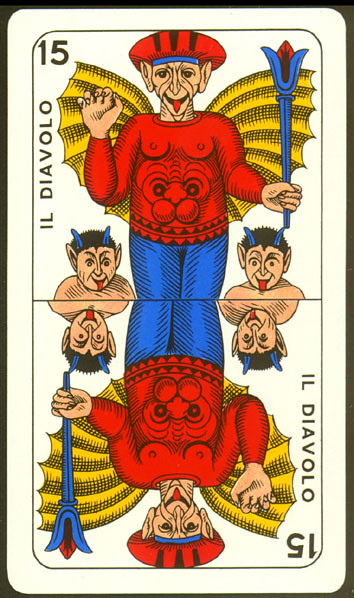This playing card features a unique and intricate design, deviating significantly from traditional playing cards. Numbered "15" in all four corners, the card is marked with the text "ILDEVOLO" written in dark brown ink, establishing its theme. The design is mirrored vertically, creating symmetry between the top and bottom halves.

At the center of the card is a prominent figure depicted as a giant man. He is waving with his right arm while holding a long, blue staff in his left. The staff is adorned with dual pointed ends and a sharp, red jewel at the top, resembling a flower, adding to the character's mystical aura. The man displays large, yellow wings that extend outward, accentuating his imposing presence. His shirt is vividly detailed with the image of a monster, characterized by oversized black eyes and cheekbones resembling those of a cat.

Flanking the central figure are two smaller demon-like creatures, each with blue horns and protruding red tongues. The demons exhibit distinct features: the one on the left sports chest hair indicated by black lines, while the one on the right appears without any. The overall aesthetic of the card conveys a demonic, otherworldly feel, enhanced by its rich details and vivid representation.